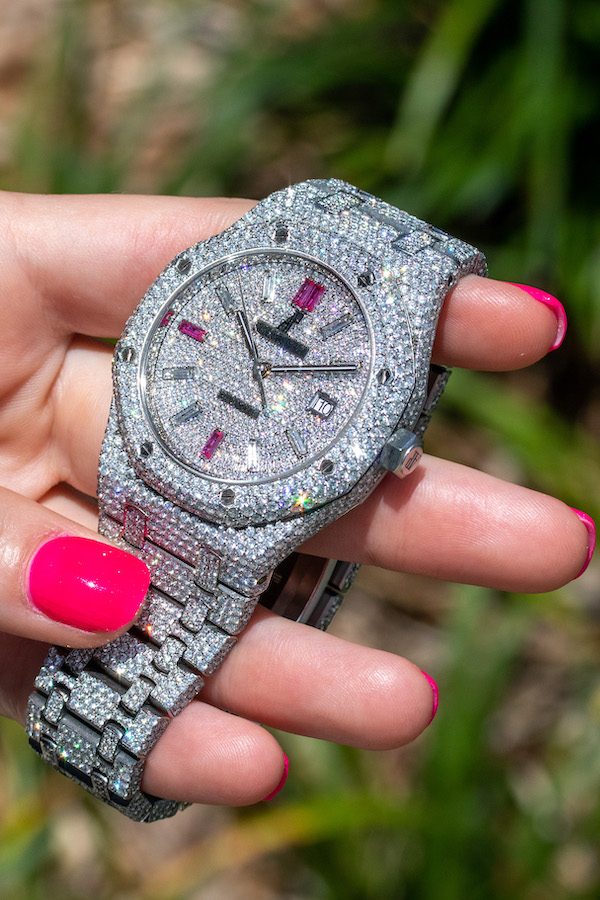In this photograph, a woman is holding a dazzling, crystal-encrusted watch with her left hand, showcasing her short, neon pink-painted nails. The silver watch is bathed in sparkling accents, featuring an analog face adorned with a mixture of clear and pink crystals. Pink diamonds mark the 12, 6, and 9 o'clock positions, while the other hours are indicated by clear or silver crystals. At the 3 o'clock position, there is a small window displaying the number 10, which likely represents the date. The silver minute and hour hands complement the watch's shimmering face. The image is taken outdoors, with out-of-focus green leaves in the background, enhancing the brilliance of the watch.